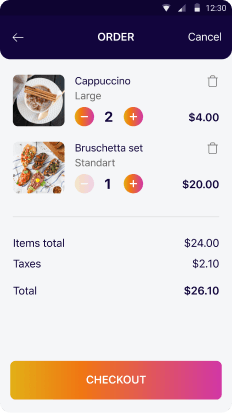**Detailed Caption:**

In this image, a screenshot taken on a cell phone captures an online checkout page for placing an order. The top right-hand corner of the screen displays essential mobile indicators: the time set at 12:30, the battery level, Wi-Fi signal strength, and cellular signal strength.

At the very top of the screenshot is the title indicating that it’s a checkout page. Below, the body of the page details the items selected for purchase. The first item listed is a large cappuccino, with a quantity of two. Each cappuccino costs $2.00, summing up to $4.00 for both. There's a small image next to the description, showing an overhead view of the cappuccino garnished with cinnamon sticks on the rim of the mug.

The second item on the list is a "Barichiteta Set," also accompanied by a tiny descriptive picture. It has a quantity of one and is priced at $20.00. 

Below the itemized list, the total costs are itemized: the subtotal for the items is $24.00, with additional taxes amounting to $2.10. This brings the final total to $26.10.

At the very bottom of the screenshot, there is a prominent, elongated checkout button, blending from yellow on the left to pink on the right. The word "Checkout" is displayed centrally in a white font.